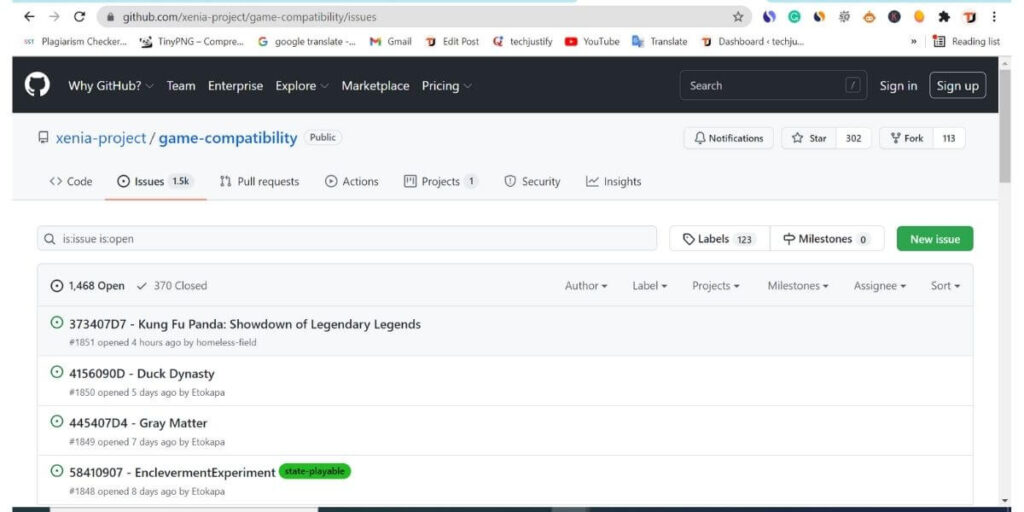This image is a detailed screenshot of a GitHub page, specifically the URL is "github.com/Xenia-project/game-compatibility/issues". The page's background is predominantly white. At the top of the page, within the browser's URL box, the specified URL is visible.

Below the URL bar, there is a line of browser bookmarks listed horizontally across the page. These bookmarks include links to various tools and sites such as "Plagiarism Checker," "TinyPNG," "Google Translate," "Gmail," "Edit Post," "Tech Justify," "YouTube Translate," and "Dashboard." 

Adjacent to the bookmark bar, at the far right, there is an option labeled "Reading List."

Beneath the bookmarks, a black horizontal banner spans the page. On the left side of this banner, an icon depicts a black cat (GitHub's logo) centered in a white circle. To the right of this icon, a series of menu options are displayed in white text: "Why GitHub?" with a downward-facing arrow, "Team," "Enterprise," "Explore" (each followed by a downward-facing arrow), "Marketplace," and "Pricing" with another downward-facing arrow. 

On the right side of the black banner, there is a search box allowing users to search within GitHub, and a "Sign Up" button for user registration.

The screenshot effectively captures the structure and elements present on the GitHub page, offering a clear view of both the navigation and the content present at the top of the site.